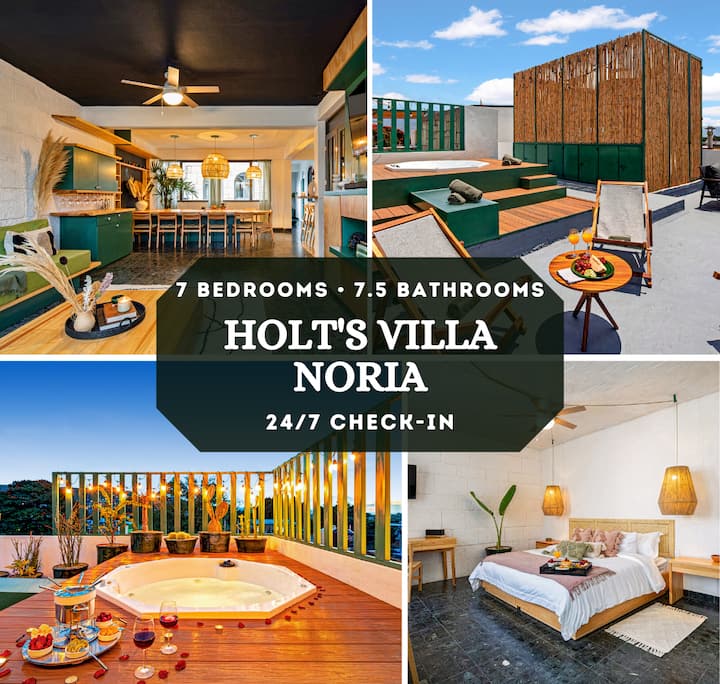This advertisement showcases Holtz Villa Noria, a luxurious villa boasting seven bedrooms, 7.5 bathrooms, and 24-7 check-in. The central image overlay provides these details, emphasizing the villa's extensive amenities. The collage of four square photographs highlights various aspects of the villa: 

- The upper left image reveals an open floor plan kitchen featuring modern elements such as white walls, a light brown ceiling fan, pendant lighting over a kitchen island, and multicolored cabinetry, creating an elegant and inviting space.

- The upper right picture captures an outdoor area with a teal-colored hot tub accessible via wooden steps, surrounded by teak furniture on what appears to be a rooftop patio. There are towels and a small table with mimosas and snacks, illustrating a perfect spot for relaxation.

- The bottom left photo provides a dusk view of the hot tub setup, adorned with string lights on a wooden railing, a pot of fondue with dipping tidbits, two wine glasses, and potted plants adding to the ambiance. The background features treetops against a blue sky.

- The bottom right image showcases one of the villa’s bedrooms, decorated with white walls, light wood furniture, and woven rattan pendant lights. The room includes a bed with white sheets and pink accents, a ceiling fan, area rugs, and potted plants, exuding a modern yet warm atmosphere.

Holtz Villa Noria offers an exquisite blend of indoor and outdoor living with its stylish and well-appointed spaces.